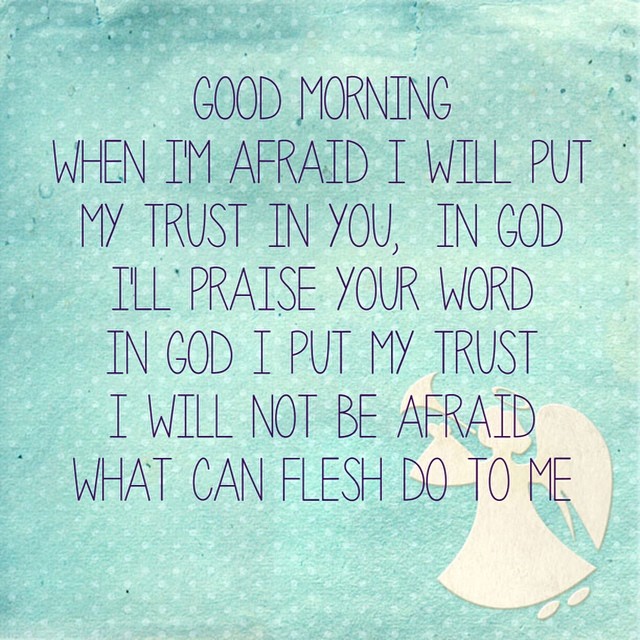The poster features a teal-blue background adorned with a pattern of lighter blue dots. Centrally positioned is a seven-line inspirational phrase in a slightly darker blue font that reads, "Good morning. When I'm afraid, I will put my trust in you, in God. I'll praise your word in God. I put my trust. I will not be afraid. What can flesh do to me?" Below the text is a cartoonish white angel, resembling a cut-out paper figure, complete with a halo and wings. The angel is depicted playing a horn or trumpet, standing upright in a white gown with two small feet visible at the bottom. The image combines elements of faith and encouragement with a whimsical, artistic design.